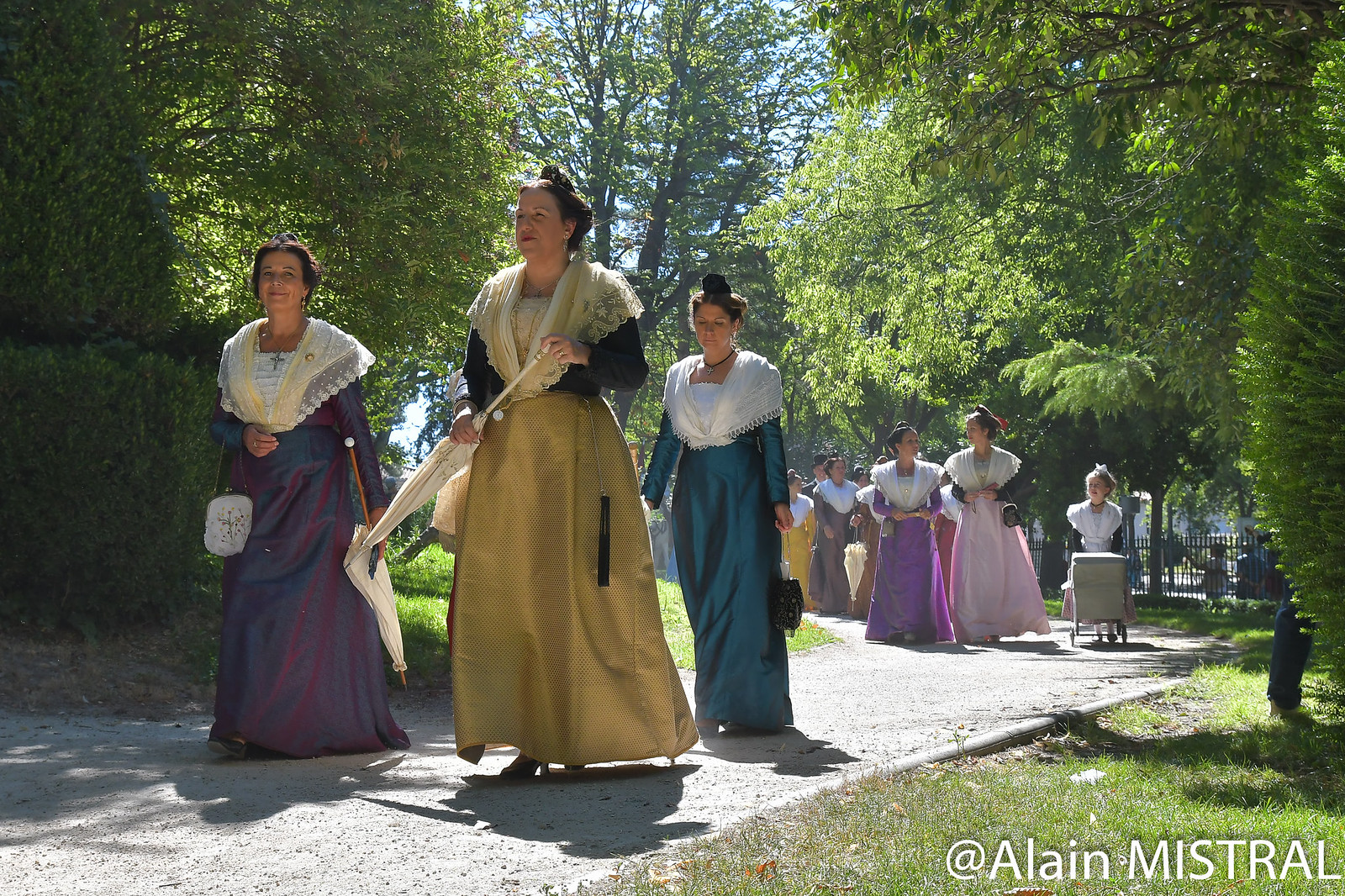In the image, a diverse group of people of different ages stroll along a gray gravel pathway, which is centrally positioned. The scene bustles with women elegantly attired in a variety of colorful dresses—shades of yellow, white, green, purple, and pink—each accessorized with white shawls, hinting at a possible celebration or a church gathering. In the foreground on the left, three women stand out: an older woman in a blue dress with a white purse, another woman in a taupe dress holding an umbrella, and a third in a blue dress with a black purse. They lead the procession, while behind them a dozen or more similarly dressed women follow. Alongside them, a young girl pushes a baby carriage. The background features verdant greenery and a light-dappled canopy of trees with patches of blue sky peeking through. A black fence runs along the far right, framing the scene. Notably, the image includes the text "© Elaine Mistral," adding an artistic touch to this vivid portrayal of communal elegance.